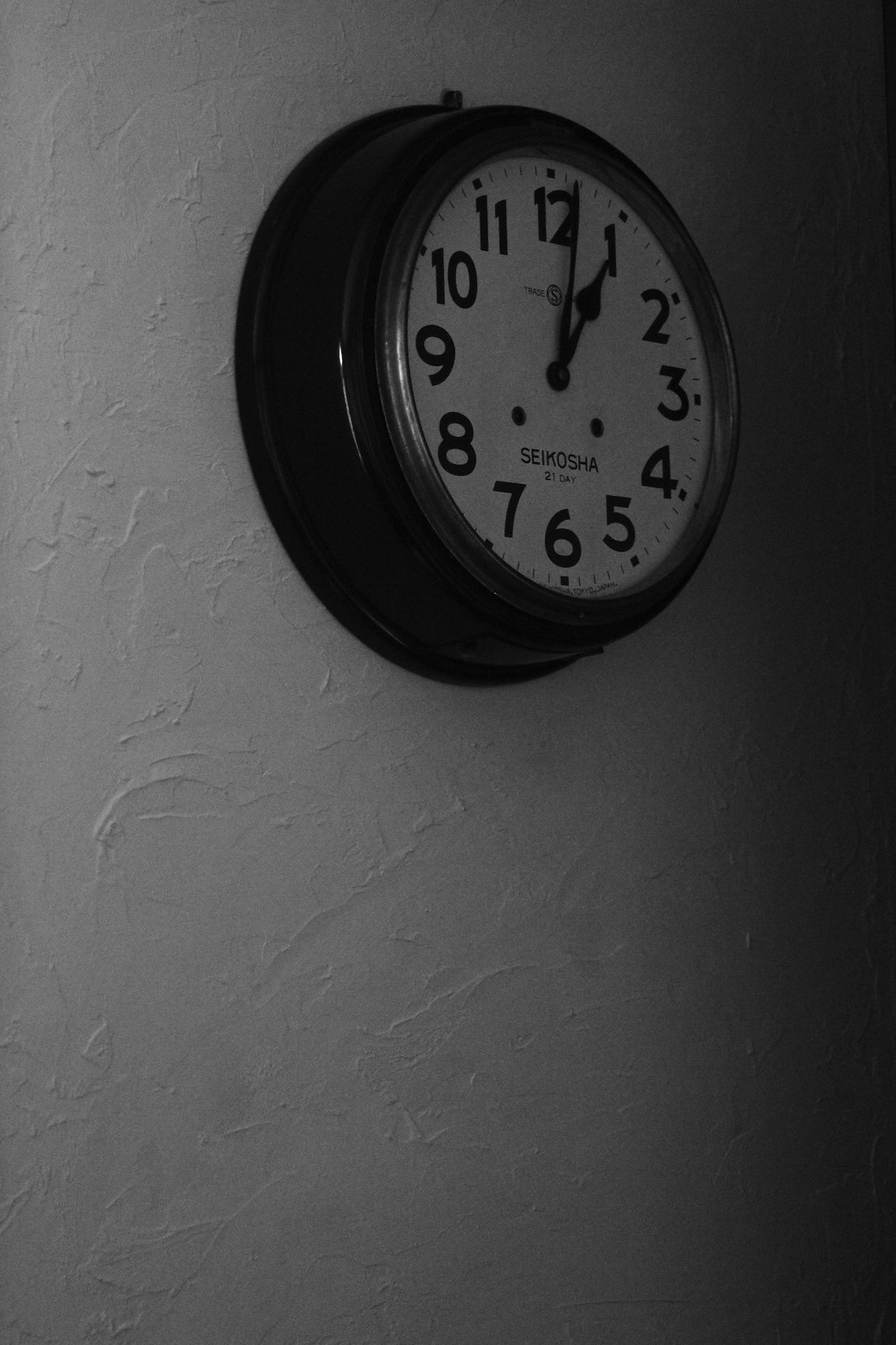The image displays a traditional Seikosha 21-day wall clock, prominently featured against a heavily textured light gray wall. The wall's deliberate splotchy texture adds a unique backdrop, almost as if the paint was applied in a swirled, pasted-on manner. The clock itself has a deep black frame, approximately 5 to 6 inches in depth, with a white face and large, easy-to-read black Arabic numerals. The short hour hand points at the 1, while the long minute hand is just past 12, indicating one o'clock. There is no visible second hand. Below the clock's hands is the brand name "Seikosha," accompanied by two small dots. Additionally, the clock features a button on top for time adjustments. The room is fairly dim, which emphasizes the wall's textured patterns and the clock's shiny black frame, making the clock's design stand out strikingly against the lighter wall. There are no other objects in the shot, focusing all attention on the clock.